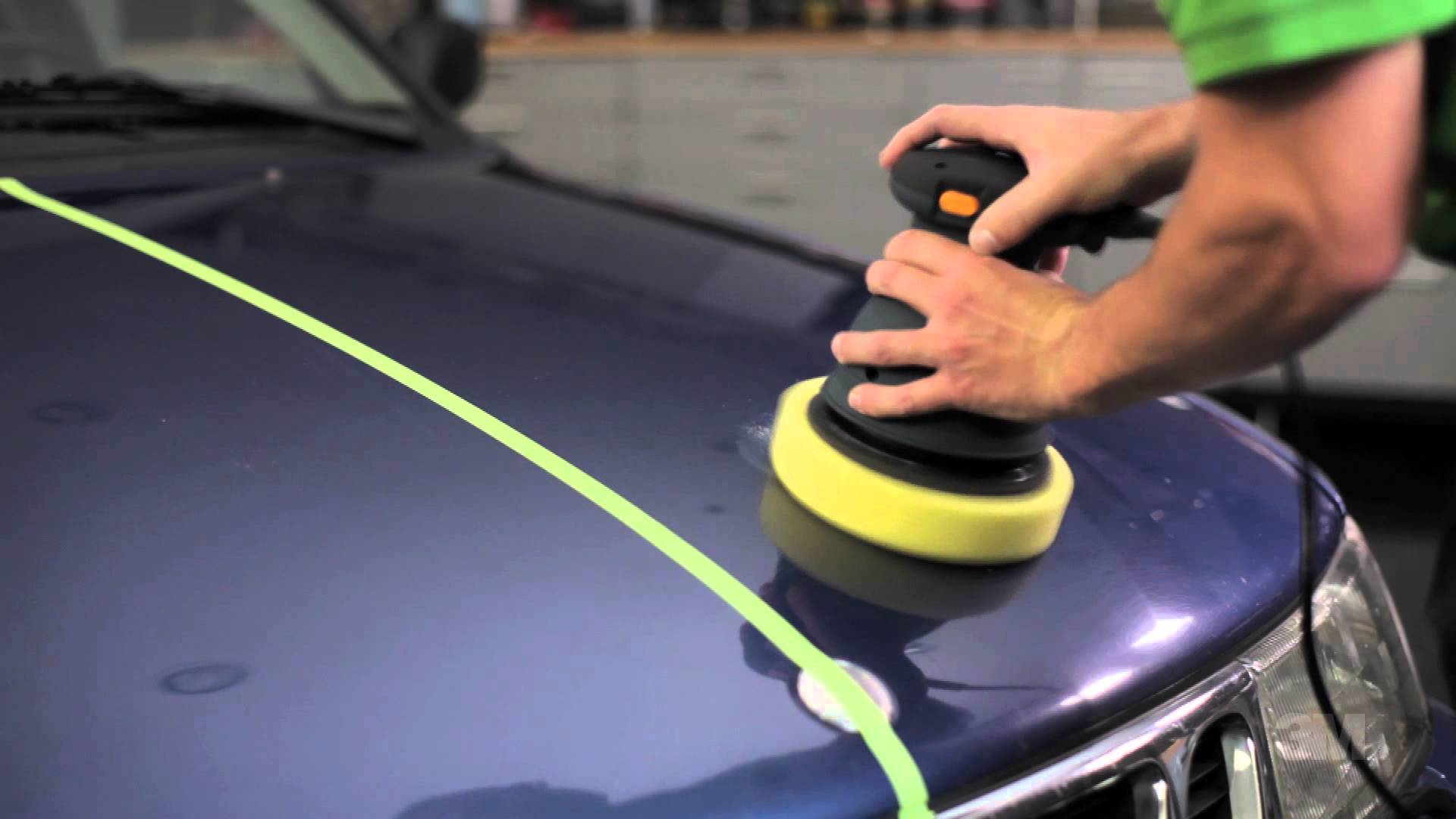The photograph captures a detailed scene inside a garage, focusing on a close-up of the hood of a navy blue car marked with a lime green stripe running down its center, which appears to be tape. On the right side, a man's well-muscled, tan arms, wearing a light green short-sleeved shirt, are seen leaning over the hood, holding a black cylindrical buffer. This machine, identifiable by its long black cord and orange button on the side, hosts a large, circular yellow foam pad at the bottom, designed to spin and polish the car's paintwork, removing scratches to make the hood shiny and glossy. In the background, well-organized white shelves reinforce the garage setting of the image.